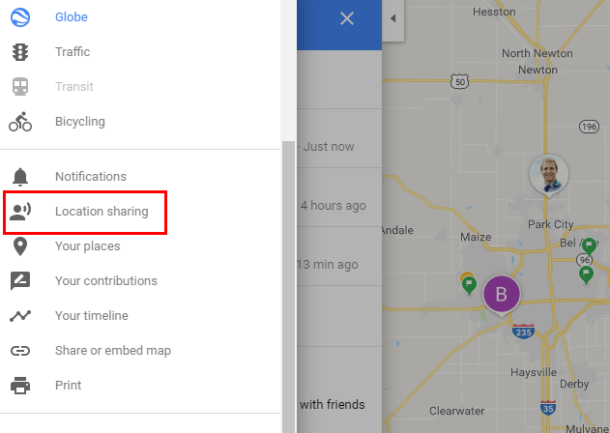The image displays a multi-layered interface featuring various informational pop-ups overlaid on a map. 

On the left side, there is a vertical pop-up window divided into two sections by a thin gray line, set against a white background. The upper section includes several icons paired with labels:
1. A blue and white circle with the word "Glow" in blue.
2. Underneath, a gray stoplight labeled "Traffic" in gray.
3. Next, a gray bus icon with the label "Transit."
4. Below that, a gray person on a bike icon labeled "Bicycling."

The thin gray line divides these from the lower section, which contains:
1. A gray bell icon labeled "Notifications."
2. A gray person icon labeled "Location Sharing."
3. A shaded box with a gray bank icon labeled "You can grade your places."
4. A gray paper with a white pencil icon labeled "Your Contributions."
5. A gray zigzag line icon labeled "Your Timeline."
6. A gray pen clip icon labeled "Share or Embed Your Map."
7. Finally, a gray print icon labeled "Print."

Behind this pop-up, there is another layer partially obscured but visible, revealing a blue border with text snippets such as "Just now," "Four hours ago," "13 minutes ago," followed by "With friends," accompanied by a white X on a blue border for exiting this section.

In the background, a partially visible map layer shows some locations in black text including "Clearwater," "Hayes," "Rail Derby," "Maize Park," "City Bell," "North Newton," "Newton," and "Heston." A purple circle with a white "B" is also visible, along with markings for highways or Interstates "35" and "235."

The overall layout suggests an interactive map interface with various user options and recent activity overlays.